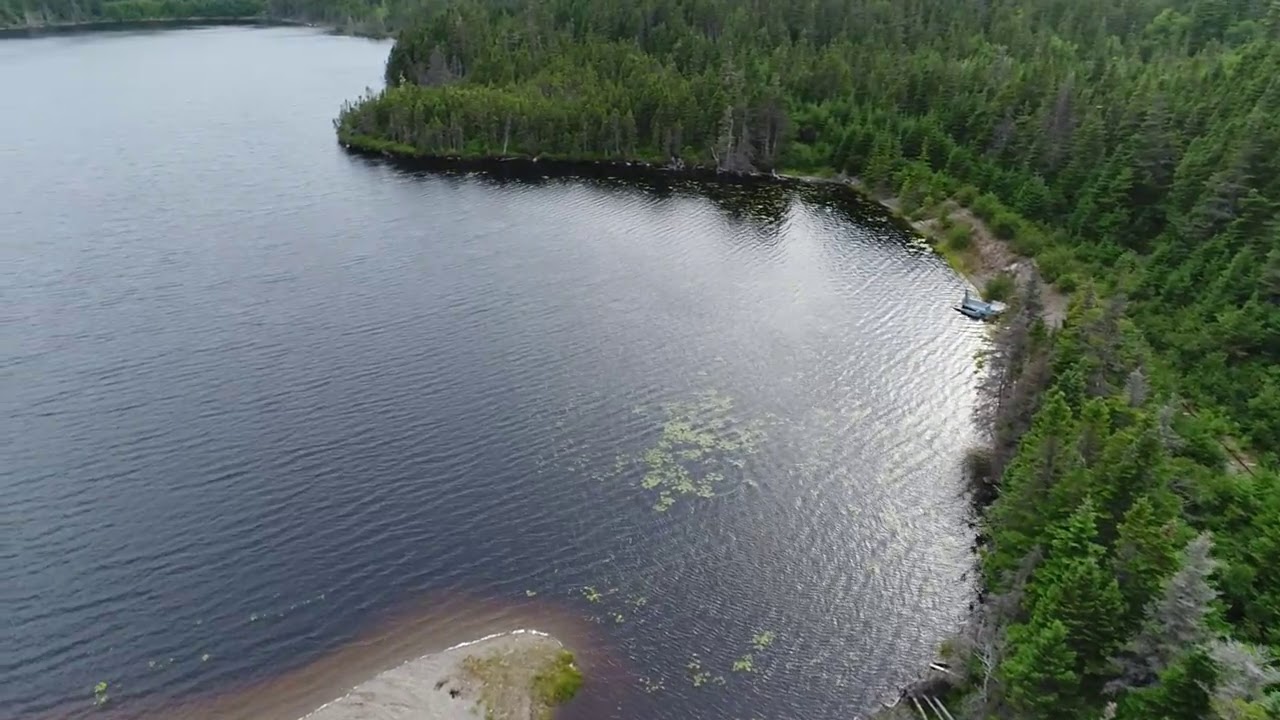This aerial color photograph captures a serene landscape in the middle of the day, showcasing a large, still body of water—possibly a lake or lagoon—set against a densely wooded shoreline. The water, a calm dark blue, holds floating light green plants and is bordered by an off-white sandbar in the bottom left corner. To the right, the land is densely populated with green pine trees interspersed with a few grey ones, and at the shoreline, several boats are pulled up near the center of the image. No people are visible in the scene, emphasizing its tranquil, undisturbed nature. The photograph, taken from above with a drone, offers a clear, detailed depiction of the natural formations and elements in the landscape.